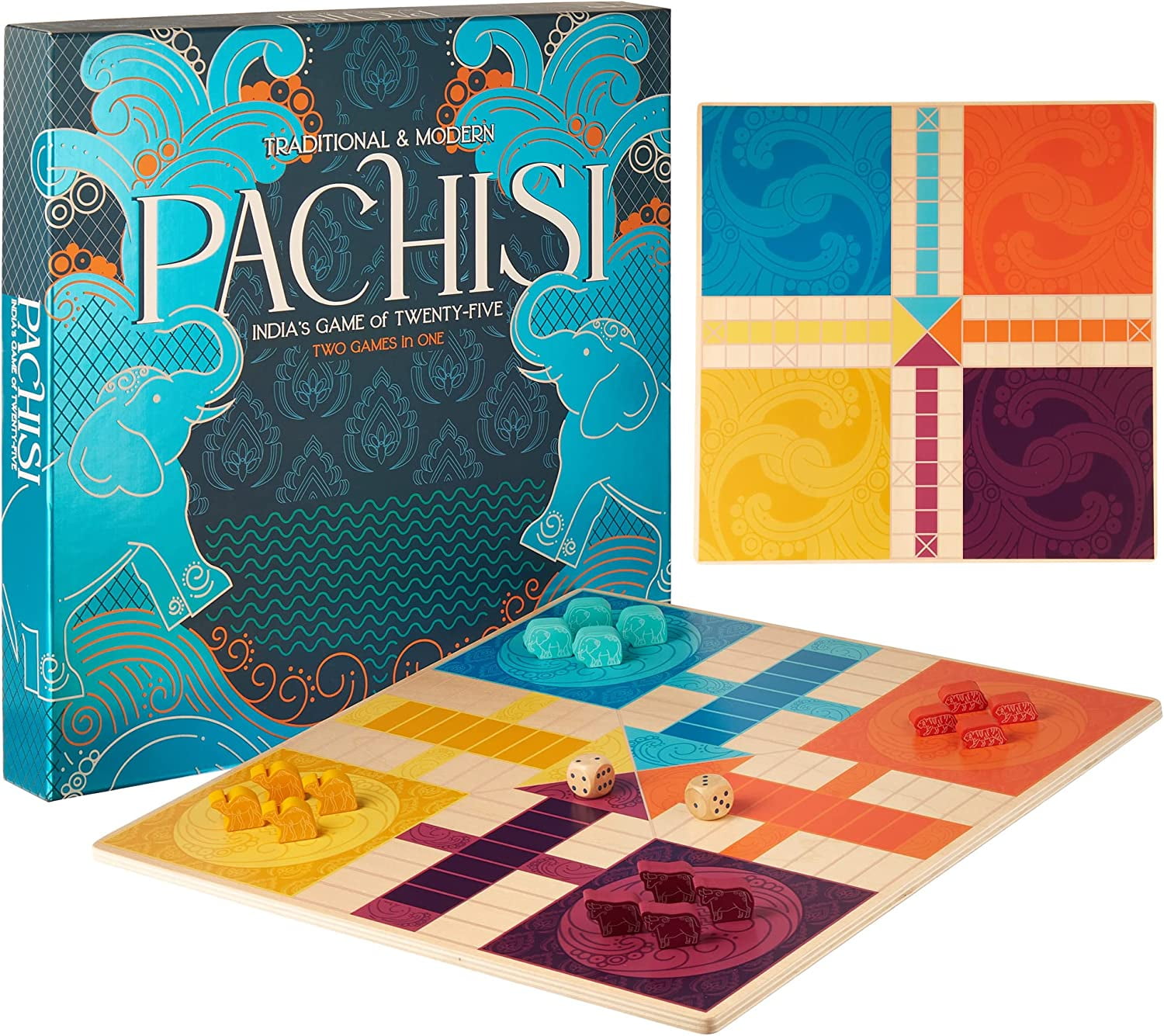The image showcases a board game called "Pachisi," also known as India's game of 25, combining elements of traditional and modern design. The box features vibrant Indian-themed artwork, including teal elephants with raised trunks and floral motifs surrounding them. The game's title and descriptions are primarily in white, with the subtitle "two games in one" highlighted in an orangish color.

The game board, displayed in the center of the image, is wooden and divided into four distinct color-coded sections: teal, red, dark red, and yellow. The board sits vertically in the top right corner, showcasing its layout clearly. Each corner hosts animal-themed game pieces: teal elephants, yellow camels, dark red cows, and orange tigers. The surface of the board appears beige or a light sand color, providing a subtle background for the vibrant pieces. Additionally, two standard six-sided dice can be seen on the board, ready for play.

The overall packaging integrates a traditional Indian aesthetic with modern gameplay elements, making "Pachisi" a visually appealing and culturally rich board game.